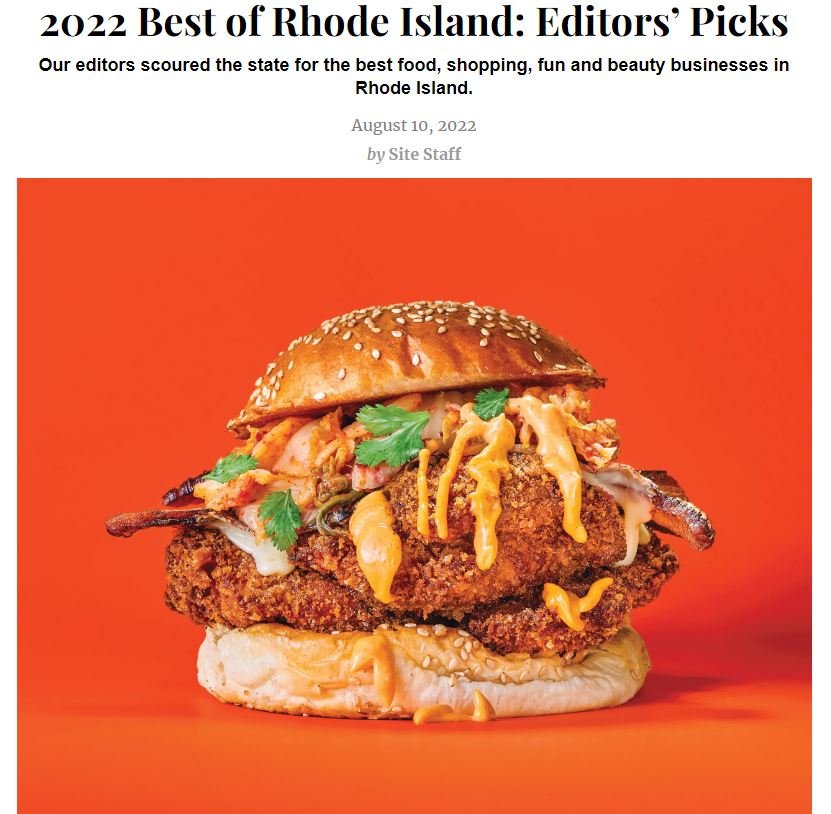This captivating image features a sumptuous sandwich that could easily be a burger, pulled pork, or even a chicken breast creation. The sandwich is adorned with sesame seeds on its golden-brown bun and is generously drizzled with an orange dressing, possibly Thousand Island. Delicate sprinkles of parsley add a touch of green, while tantalizing strips of bacon peek invitingly from the sides. The vibrant orange background enhances the visual appeal of the sandwich, making it the focal point of the image.

At the top of the picture, there is a heading that reads "2022 Best of Rhode Island: Editor's Picks." Directly beneath this, in smaller black font, it states, "Our editors scoured the state for the best food, shopping, fun, and beauty businesses in Rhode Island." This announcement is further detailed with a timestamp "August 10th, 2022 by Site Staff," with "Site Staff" distinctively spelled as S-I-T-E. The date and authorship are presented in a subtle gray font.